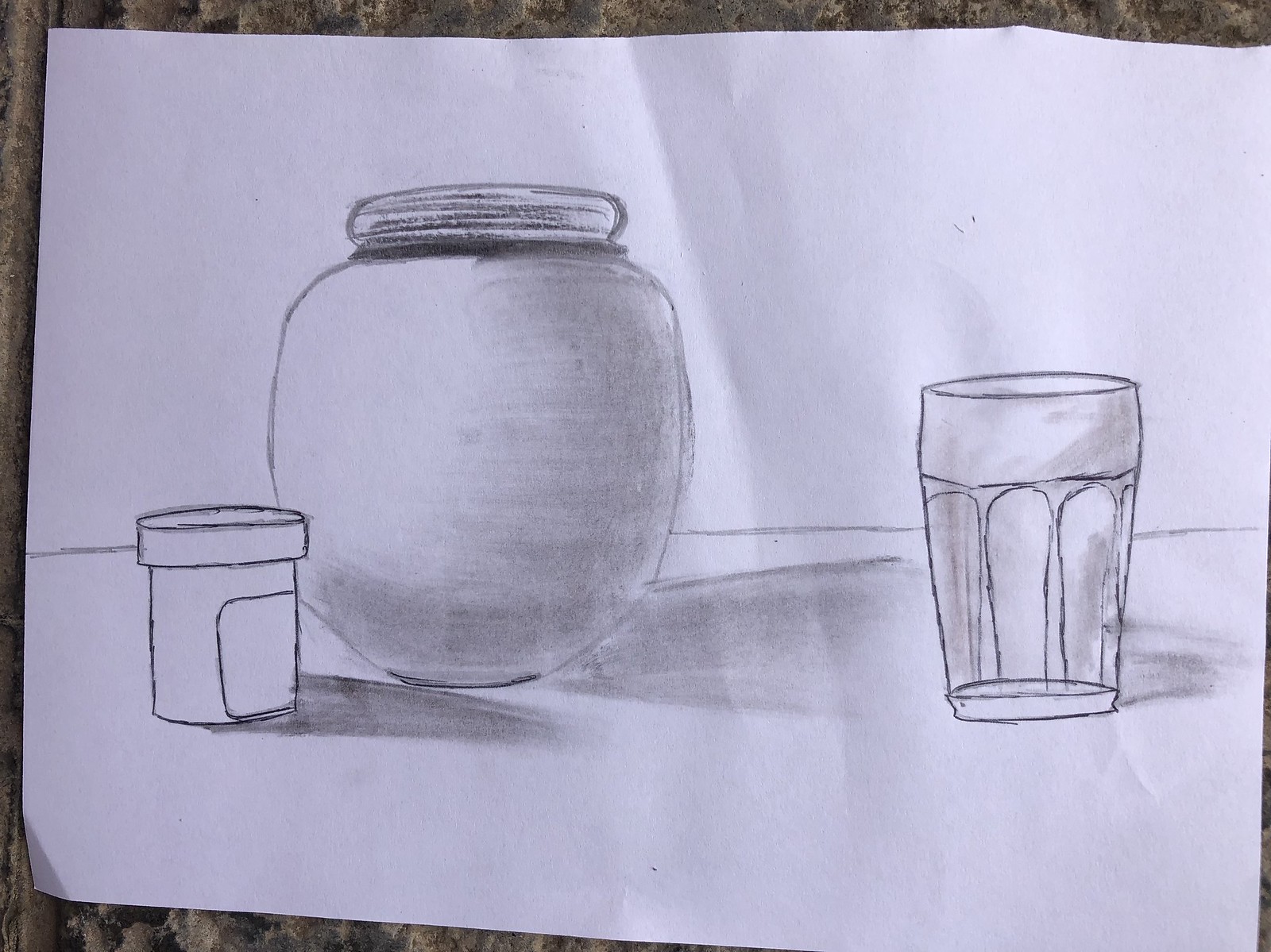This is a detailed pencil drawing on a slightly crinkled, white piece of paper, positioned vertically. The scene features a large, round jar with a lid in the center, slightly towards the left. To the bottom left of the jar is a cylindrical medicine bottle with a safety cap and a blank label. On the right side of the image, there's an intricately detailed glass with three arches, suggesting it’s made of clear crystal. Shadows cast by the jar, medicine bottle, and glass add depth to the sketch. A horizontal line runs halfway across the drawing, indicating the edge of a table or countertop, possibly dark and marbled. The background reveals a rough, possibly brown surface, resembling carpet or a wall. The shading techniques, primarily in gray and some black, enhance the three-dimensional feel of the objects.